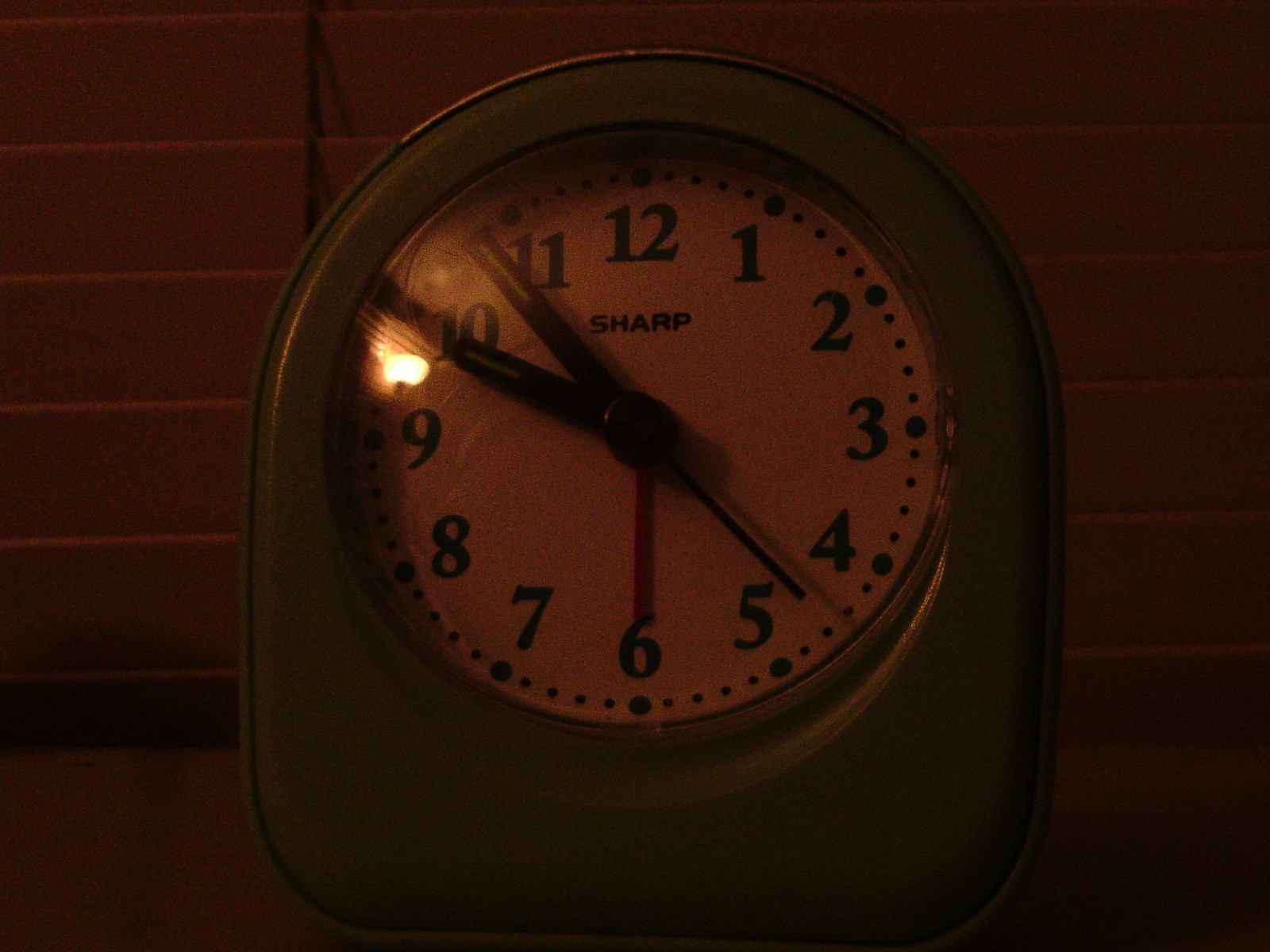This eerie photograph captures an old-fashioned clock positioned in front of partially open blinds. The clock face displays the time as 9:54, likely PM, given the surrounding darkness. In the upper right corner of the clock’s glass, there is a visible reflection of a light source, adding to the photo's mysterious atmosphere. The clock appears to be an alarm clock, distinguished by two additional hands set at different positions, possibly indicating the alarm time. This finely detailed image evokes an uncanny sense of anticipation and stillness.